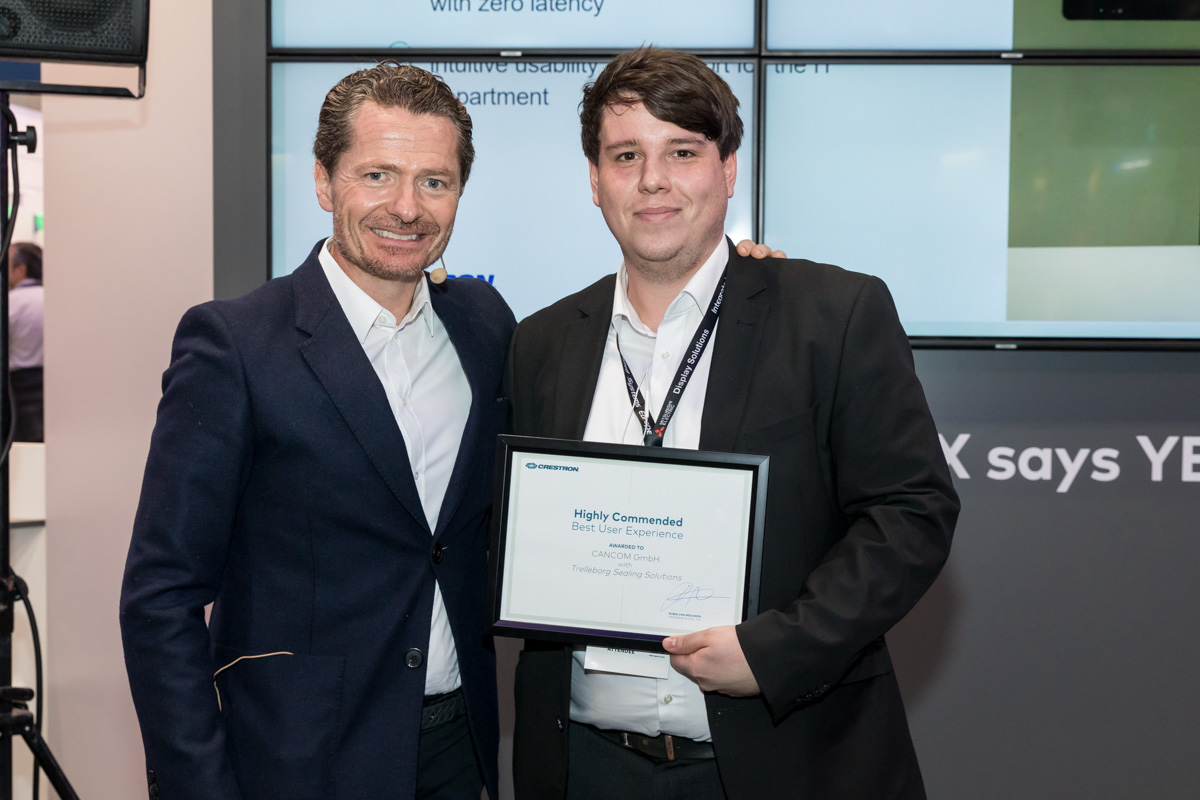In this photograph taken at a business conference, two men are posing together. The background features a wall comprised of several wide, rectangular TV screens displaying portions of a PowerPoint presentation, with discernible text fragments including "apartment," "disability," "zero latency," and "with zero latency." The man on the left, appearing to be in his forties with graying brown hair and some facial hair, is dressed in a white button-up shirt, a blue jacket, and black pants. He has his arm around the shoulder of the man on the right, who looks younger, with brown hair and white skin. The younger man is wearing a white button-up shirt, a black suit jacket, and black pants. He is holding a framed award that reads "Highly Commended Best User Experience," although the finer details are too small to make out clearly. Their mutual gesture of camaraderie suggests a celebratory moment. In the backdrop, additional elements include portions of a beige wall, a possible partial speaker on a stand, and another person wearing a white shirt and black pants, indicating a gathering of people.